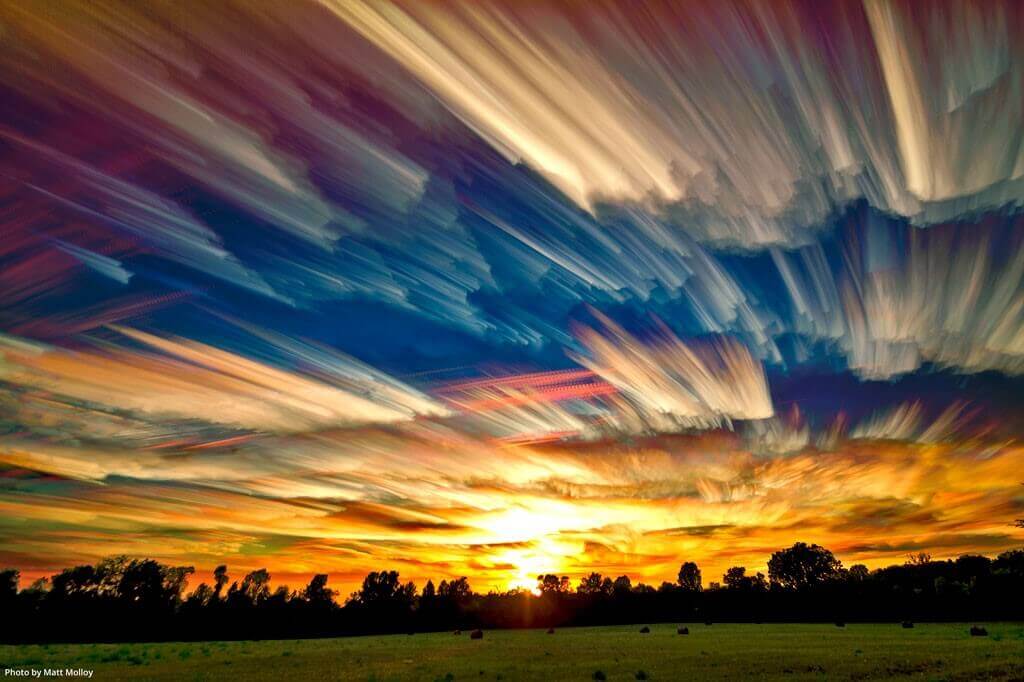This striking, animated image, labeled "photo by Matt Malloy" at the bottom left, showcases a vibrant and dynamic sunset scene. Dominating the composition, the sky spans approximately three-fourths of the image, transitioning from deep blue at the top through layers of orange, red, and yellow hues suggestive of a timed photo capturing the setting sun. Streaks of white light create a sense of motion and fading into darker blue shades towards the upper edge. Below this vibrant sky is a silhouette of trees and an open field, with details like indistinct figures or bales of hay blending into the dark green grass. The high contrast between the blackish tree outlines and the vivid colors above emphasizes the sunset's dramatic effect.